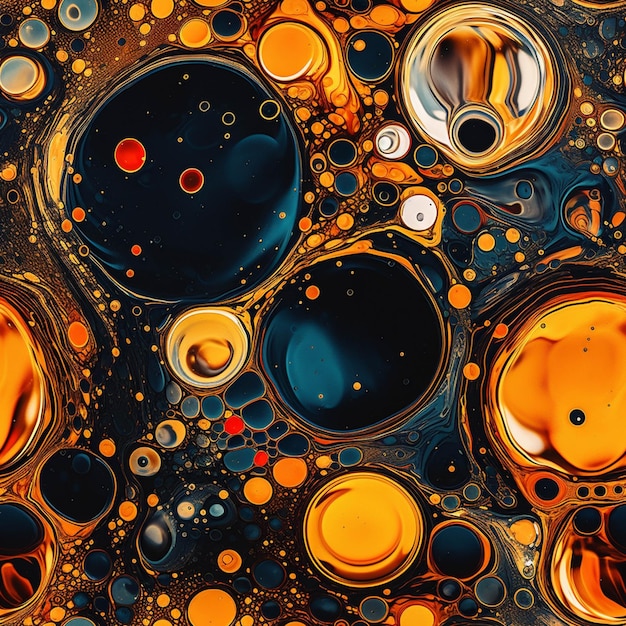The image is an abstract painting that captures a vivid and surreal scene resembling a universe of bubbles or spheres in a liquid-like medium. It features numerous bubble-shaped spheres of varying sizes and shapes, with each bubble displaying a range of bright and bold colors including blue, yellow, red, orange, and some black and white. The spheres appear to float, giving a sense of depth and movement, as if suspended in water or a mystical outer space environment. Notably, some of the blue spheres contain smaller bubbles within them, enhancing the layered effect. A striking silvery bubble stands out in the top right, adorned with reflections of orange, light blue, and white. Darker spheres, reminiscent of containing miniature universes, add to the painting's ethereal and otherworldly feel. One sphere in the bottom right intriguingly resembles a fish, albeit with digital artifacts, suggesting possible AI generation. The overall composition is an intricate and highly detailed fusion of colors and forms, evoking a sense of wonder and abstract beauty.